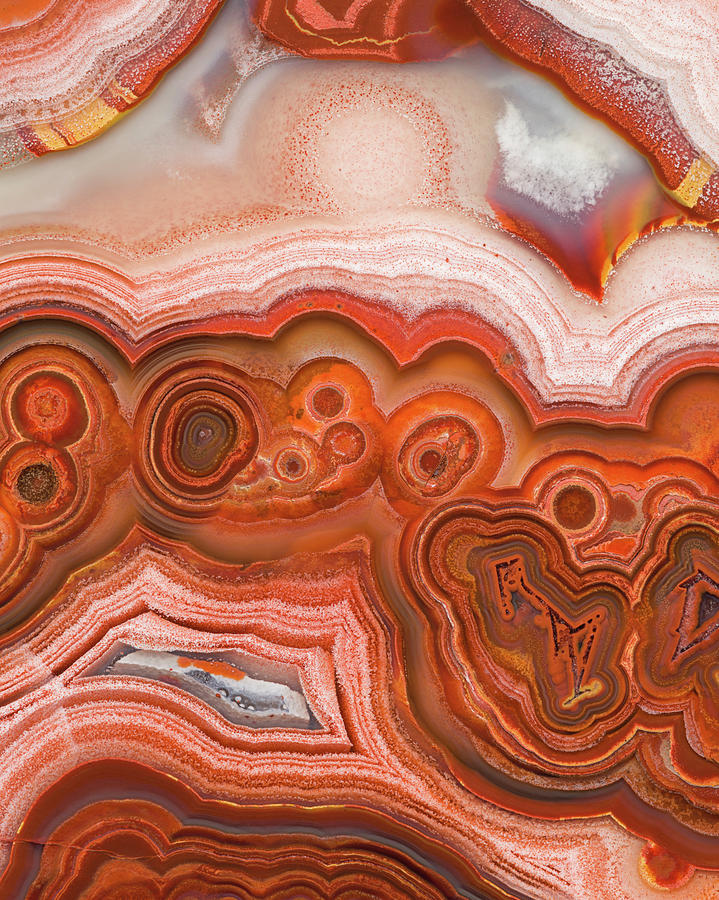The image showcases a stunning and intricate design characterized by swirling colors that resemble a polished piece of rock quartz. Vibrant reds, oranges, yellows, pinks, and whites dominate the composition, with accents of blue and dark brown adding depth and contrast. The upper third of the image features lighter hues, akin to sand, while the lower portions are rich with various shades of red, from light to dark. The design is composed of circle-like and wave-like patterns, which evoke the appearance of cells or even a distant planet's surface. These elements create a complex and mesmerizing piece of art that, despite having no distinct pattern, forms a harmonious and captivating visual experience.